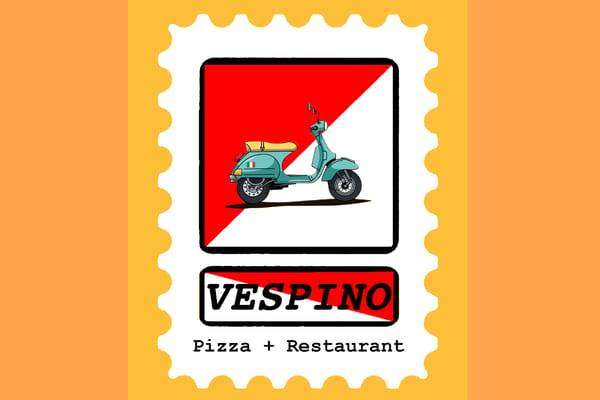This is a detailed digital drawing designed for advertising a pizza restaurant named "Vespino." The overall background is orange, with a central block that is a lighter shade of orange, bordered by a white area resembling the edge of a postage stamp with notched edges. In the center of this stamp-like border is a square divided diagonally into red on the top left and white on the bottom right. Positioned centrally within this square is a green Vespa motor scooter with a yellow seat, headlight, and handlebars. Below the scooter, there is an oblong circle with the word "Vespino" written inside, also divided diagonally into red and yellow. Just beneath this, in black text, it says "Pizza Plus Restaurant." The color scheme consists of red, white, black, orange, and yellow, reinforcing its purpose for eye-catching restaurant advertising.